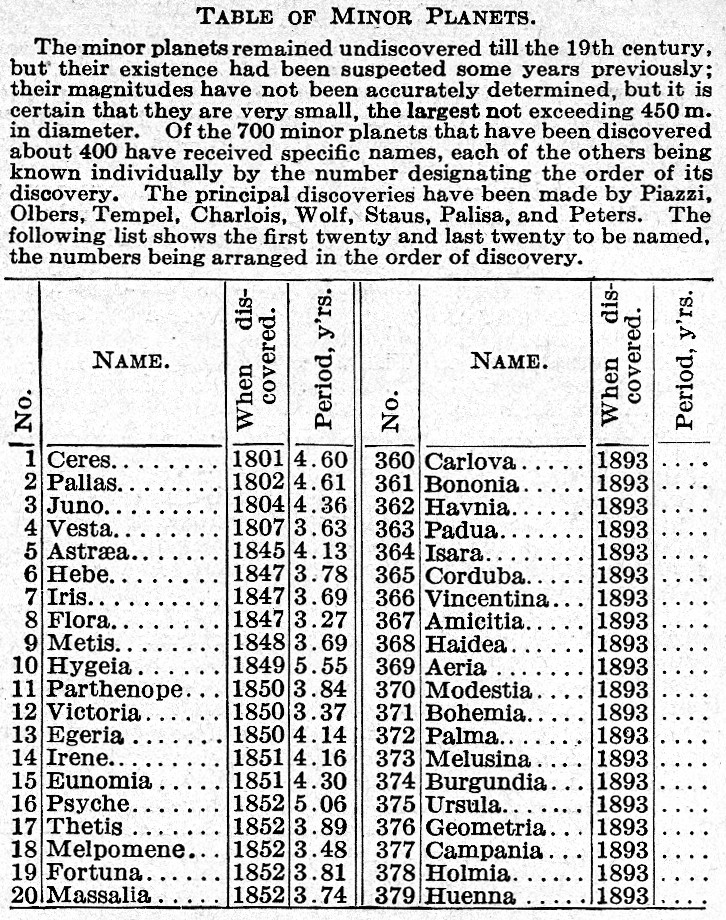The image is a detailed snippet from a reference book or textbook featuring a section titled "Table of Minor Planets," centered at the top. Below this heading, there is a paragraph that explains the history and discovery of minor planets. It states that minor planets remained undiscovered till the 19th century, though their existence was suspected earlier. Their magnitudes have not been accurately determined, but it is certain that they are very small, with the largest not exceeding 450 meters in diameter. Of the 700 minor planets discovered, about 400 have received specific names, while the others are known by the number designating their order of discovery. The key discoveries were made by astronomers such as Piazzi, Olbers, Tempel, Charlois, Wolff, Staus, Palisa, and Peters. Following the paragraph, there is a table with several columns and multiple rows, all in black text against a white background. It displays the first 20 and last 20 named minor planets, categorized by number, name, date of discovery, orbital period, and years since discovery, arranged in the order of their discovery.